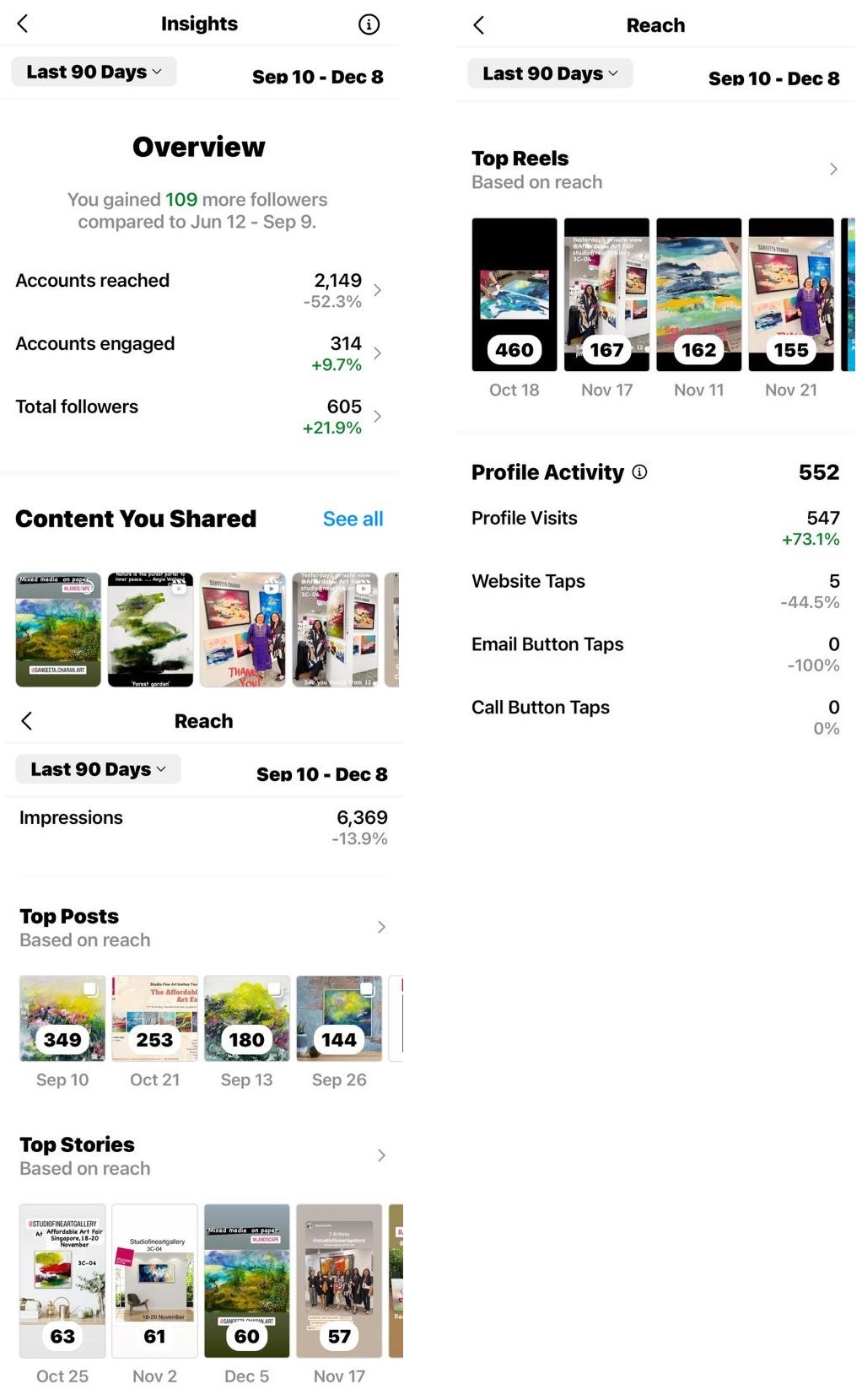The image consists of three detailed screenshots from a smartphone or website analytics dashboard, each providing insights on user engagement over a specific time period. The screenshots are laid out with one on the top left, one on the top right, and one on the bottom left.

1. **Top Left Screenshot: Overview of Insights**
   - **Header:** Includes a left arrow and the title "Insights."
   - **Date Range:** Last 90 days, from September 10th to December 8th.
   - **Section Title:** "Overview."
   - **Follower Growth:** "You gained 109 more followers compared to June 12th to September 9th."
   - **Metrics:**
     - **Accounts Reached:** 2,149, a decrease of 52.3%.
     - **Accounts Engaged:** 314, an increase of 9.7%.
     - **Total Followers:** 605, an increase of 21.9%.
   - **Design:** All text is black on a white background.

2. **Top Right Screenshot: Reach Insights**
   - **Header:** Includes a left arrow and the title "Reach."
   - **Date Range:** Last 90 days, from September 10th to December 8th.
   - **Top Views Based on Reach:**
     - Screenshots of posts/stories with views displayed in white rectangles:
       - 460 views on October 18th
       - 167 views on November 17th
       - 162 views on November 11th
       - 155 views on November 21st
   - **Profile Activity Metrics:**
     - **Total Profile Visits:** 552
     - **Profile Visits:** 547, an increase of 73.1%.
     - **Website Taps:** 5, a decrease of 44.5%.
     - **Email Button Taps:** 0, a decrease of 100%.
     - **Call Button Taps:** 0, no change (0%).

3. **Bottom Left Screenshot: Reach and Impressions**
   - **Header:** Includes a left arrow and the title "Reach."
   - **Date Range:** Last 90 days, from September 10th to December 8th.
   - **Impressions:** 6,369, a decrease of 13.9%.
   - **Top Content Metrics:**
     - **Top Post (based on reach):** Four posts with dates and reach numbers displayed in white rectangles.
     - **Top Stories (based on reach):** Four stories with similar formatting, including reach numbers in white rectangles and dates below each.

All screenshots share the same clean, white background, and are designed for easy readability and comparison.